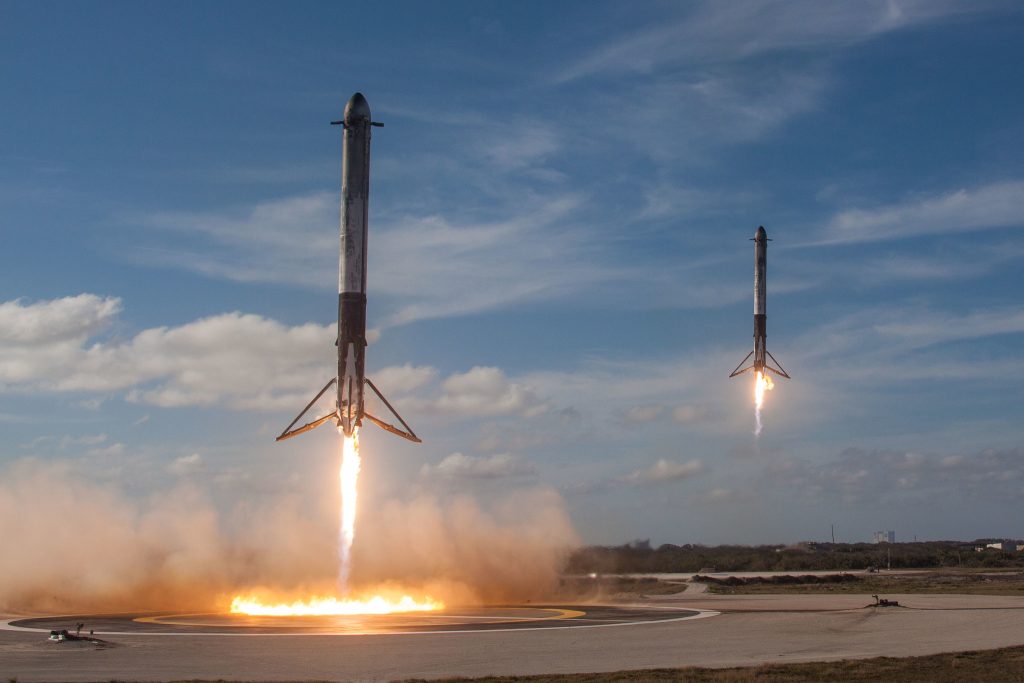This outdoor daytime photograph captures the dramatic moment of two rockets taking off into the sky. The foreground features a large metal rocket with a straight cylindrical form, identifiable by its two protrusions near the nose and four triangular fins at its tail, set against a background of billowing smoke and vibrant flames at the base, indicating its imminent ascent. Launching from a pad marked with circles, this rocket stands prominently on the left side of the image. To its right, or behind it, appears a second rocket, similar in shape but seemingly smaller due to its greater distance from the camera. This rocket also emits fire from its bottom as it climbs skyward. The clear blue sky, dotted with bright white clouds concentrated mostly to the left, frames the scene, while hints of green trees line the horizon in the background, providing a serene contrast to the powerful, fiery spectacle of the rockets' launch.